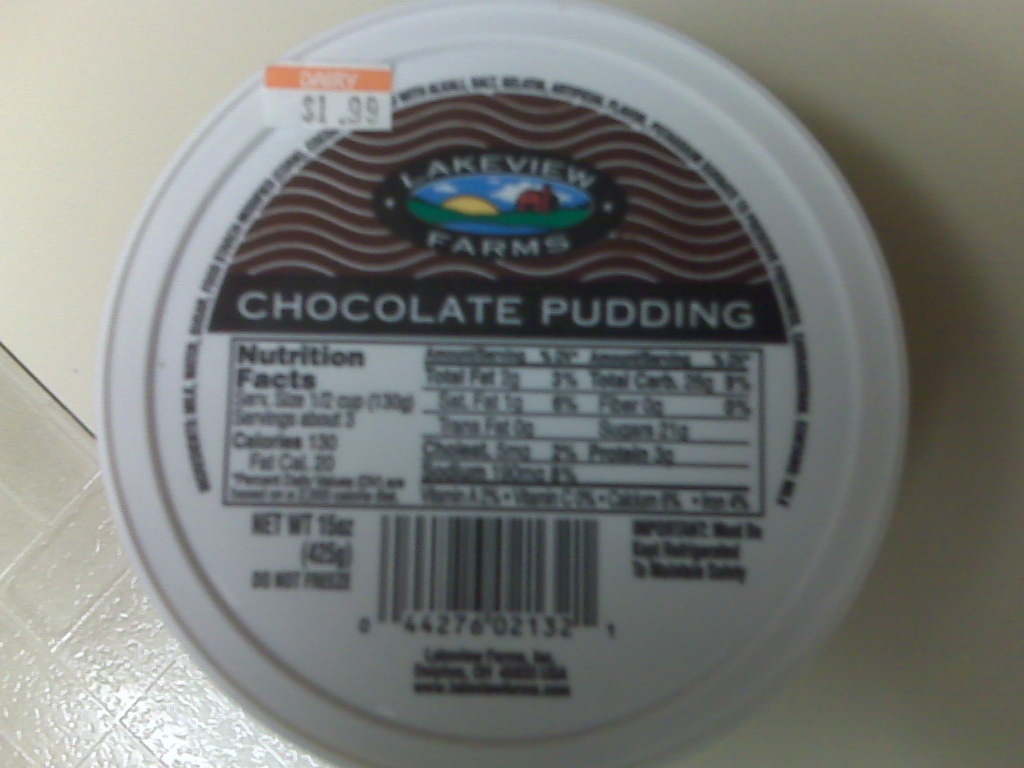This close-up photograph, taken from above, captures a blurry yet detailed view of a Lakeview Farms Chocolate Pudding cup positioned on a cream-colored counter. Dominating the image is the white, lidded container, prominently displaying a price sticker marked with an orange stripe reading "grocery $1.99." The lid itself features a detailed logo of Lakeview Farms, illustrating a picturesque scene with a bright sky, a red barn, a yellow sun, clouds, blue pond, and green grass, all framed by squiggly brown lines presumably indicating the chocolate flavor. The words "Chocolate Pudding" are boldly printed in white font beneath the logo. The tub, which holds a net weight of 15 ounces, includes a nutrition facts label below the main graphics, though the text is largely unreadable due to the photograph's blurriness. The bottom portion of the container also displays a barcode. The surface beneath the cup hints at white tile or linoleum flooring, reflecting light in parts.